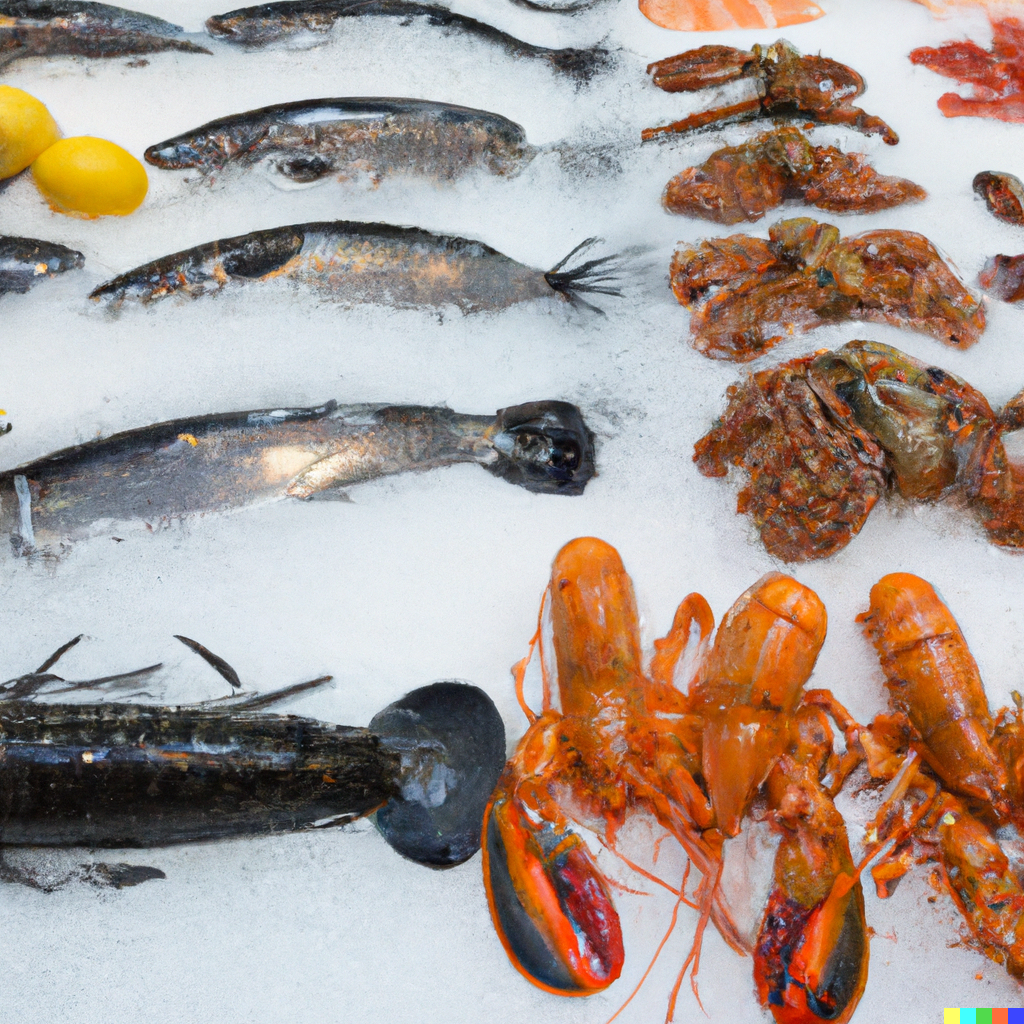This photograph captures a meticulously arranged display of various seafood, set indoors with a stylish, photographic backdrop. The seafood is packed on ice, with three vibrant orange lobsters prominently featured in the foreground, their heads angled downward. To the left of the lobsters lies a black fish, its tail extending towards them. Just above the lobsters, three orange crabs are grouped together. To the left of the crabs, four silver fish with black tails are arranged. A pair of lemons can be found in the upper left corner, adding a splash of color. Tucked into the upper right corner is a hint of red, possibly crab claws. The image also contains a small graphic at the bottom, consisting of yellow, blue, red, and dark blue bands, but no additional text.